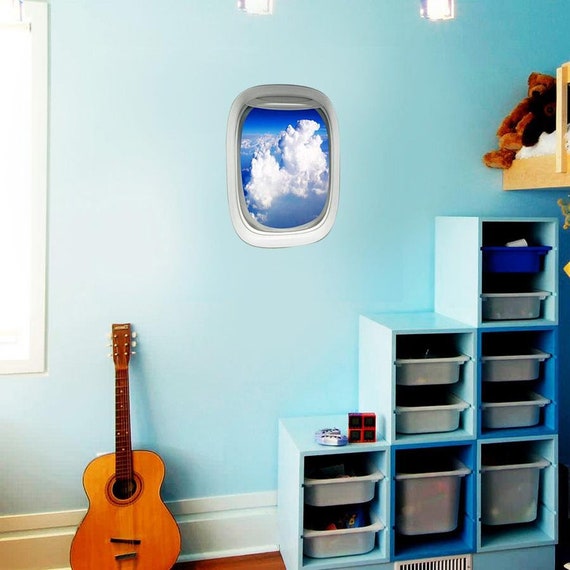This image depicts a domestic bedroom characterized by sky-blue walls and an eclectic mix of decor and furniture. Dominating the visual is a digitally added image that gives the illusion of an airplane window occupying the center of the wall. The window frame is silver and showcases a deep blue sky dotted with cumulus clouds, enhancing the surreal atmosphere of the room. 

To the left edge of the photograph, a border of bright light likely indicates another window bringing natural light into the space. Below this, an acoustic guitar with a light wooden body and a dark neck leans against the wall on a section of wooden painted floor peeking out from beneath the furniture.

On the right side, there's a complex storage solution consisting of a series of cubby-like compartments painted to match the walls. The compartments are organized in a stepped arrangement and filled with various gray and blue plastic trays.

Additionally, the top portion of a bunk bed with a light wooden frame is visible in the photo's top right corner, adorned with a stuffed animal that looks like a teddy bear. The framework of the bunk bed includes two small light bulbs near the top, contributing to the soft ambiance of the room. 

Overall, the image merges mundane domestic elements with an unusual digital addition, creating a visually intriguing scene without any explicit context or human presence.